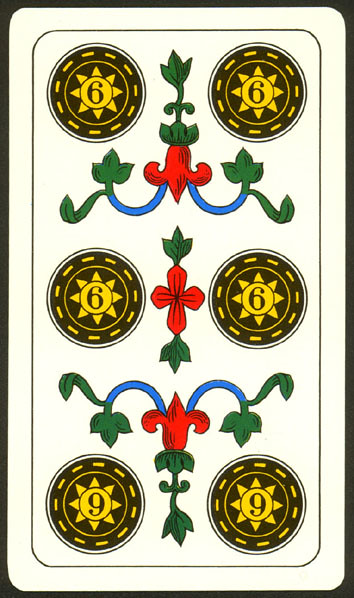This is a color drawing resembling a playing card, set against a white background with a thin black border. The card is organized into three rows, each containing two black poker chips, making a total of six poker chips, placed in the top corners, middle, and bottom corners of the card. Each poker chip features a detailed design with dashed yellow lines encircling a yellow circle that contains a sun-like figure. Inside this yellow sun, there is a black number six.

The poker chip designs are further embellished with unique symbols and colors. The top two poker chips have what appears to be a mustache-like figure with green, red, and blue hues. The middle two display a cross-like symbol in red. The bottom two have an upside-down mustache design, similar in color to the top symbols.

Additionally, green vines are interspersed among the poker chips. These vines, some transitioning into blue and red sections, contribute to the ornate design. In the center of the card, there is a red rose-like form resembling a cross, flanked by three-leafed leaves emerging from the top and bottom. The overall composition combines plant motifs and geometric shapes, and the balance of elements creates a rich, intricate visual effect.